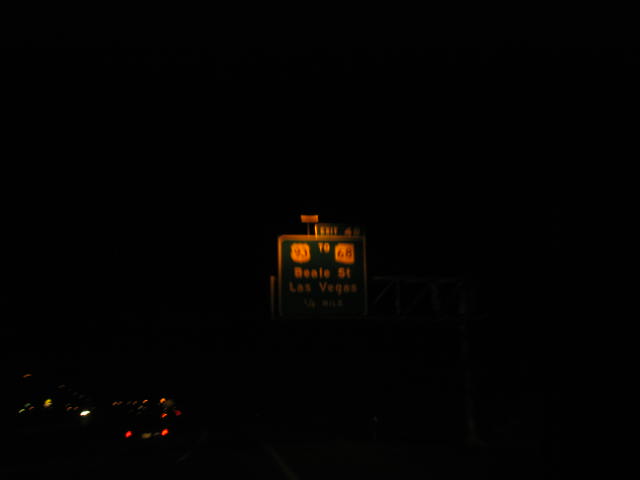This is a nighttime photograph taken from a highway, featuring a prominently displayed green highway exit sign for Beale Street in Las Vegas. The sign, which is blurred but still legible, indicates the routes 93 and 68. The exits are partially visible with the word "exit" at the top. Surrounding the sign is a dark background, with the only illumination coming from the headlights and taillights of several cars situated in the lower left-hand corner of the image. The rest of the photo is predominantly black, emphasizing the central highway sign.